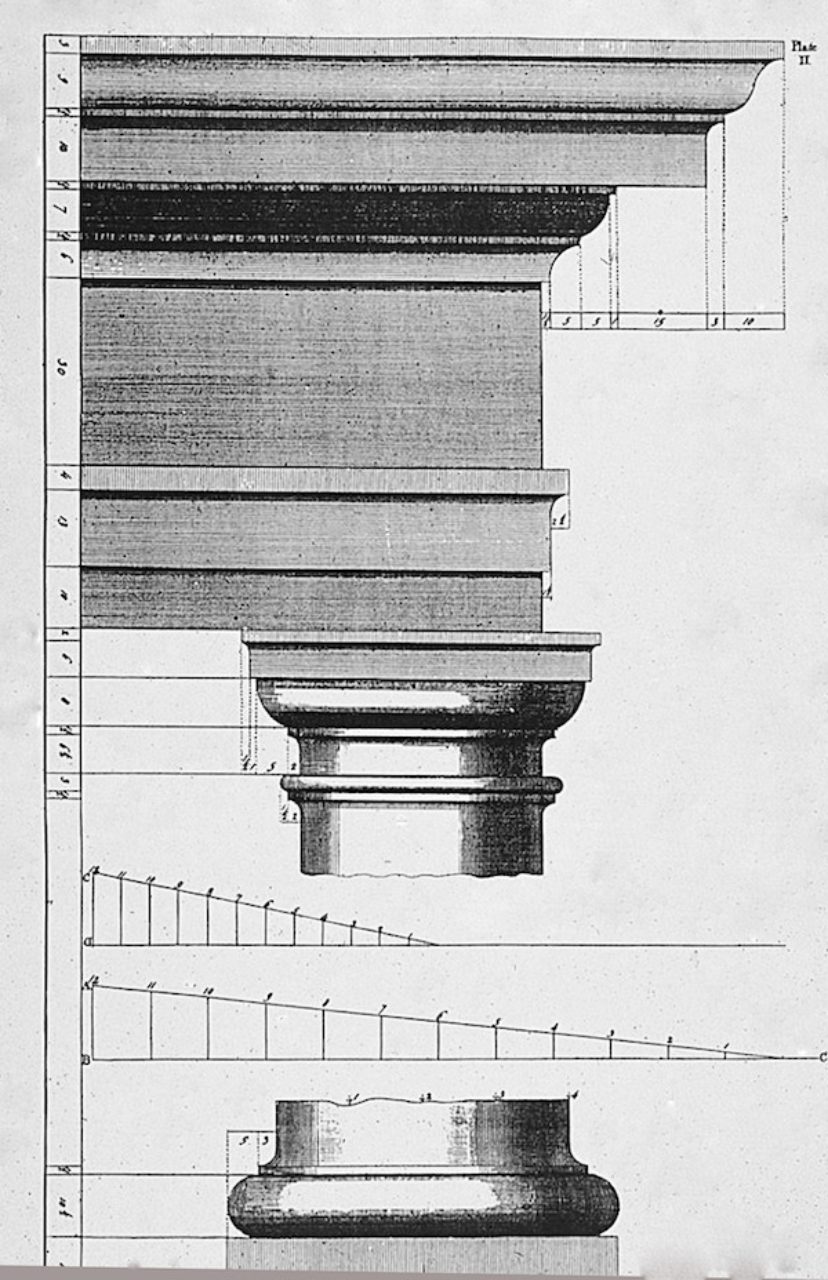This is a detailed, pencil-sketched mechanical drawing that appears to depict architectural elements such as crown molding and a cylindrical column, possibly intended for a home, museum, or library. The black and white diagram reveals a section of crown molding on the right, characterized by a swooping lip that mirrors classic ceiling designs. On the left, there’s a vertical strip featuring numerous numbers and pencil markings, likely denoting measurements in centimeters or millimeters. The drawing includes detailed representations of wood grain, various pencil marks, and measurement lines, with no explicit scale provided. The illustration also shows a column split in half, with angles between the two halves and additional measurements specifying areas that might feature lathe work, highlighting variations in diameter. The precision and elegance of the drawing suggest it was likely created by an engineer or machinist specializing in woodworking. The overall composition, square figures, and block figures supporting the main design, provide a clear and sophisticated blueprint of how these architectural features should be constructed.